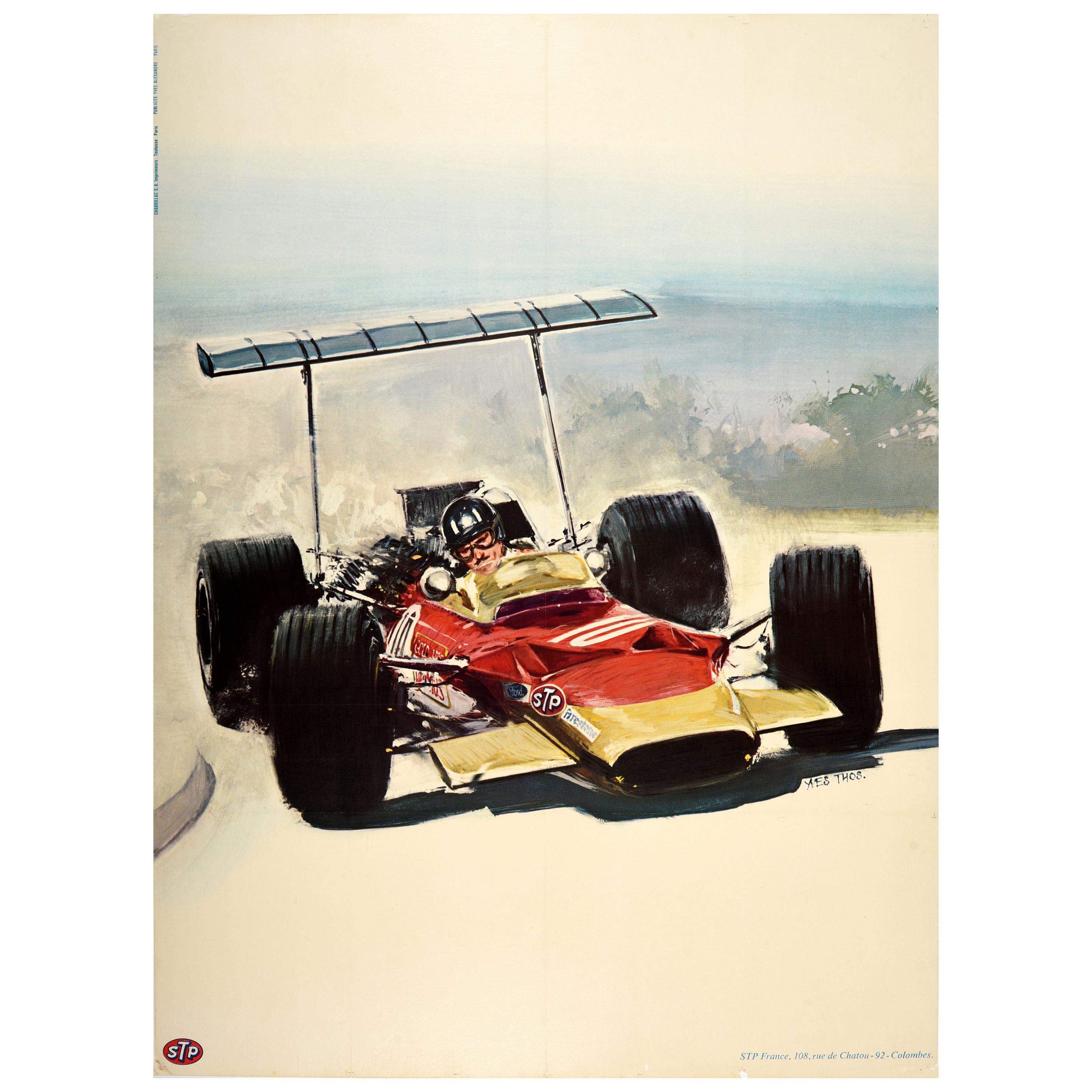The illustration depicts a vintage Formula One race car navigating a corner on a dirt track. The car is an open-top, one-seater vehicle, predominantly colored in gold, red, and white. It features a high-mounted spoiler and a fin at the back for downward pressure. The race car has four large black tires, with the number "10" displayed in black on a white circle on the lower left side, along with the logo "STP". The driver, a man with lighter skin, is equipped with a black helmet, brown goggles, and a mustache. He appears focused as he grips the wheel. The background transitions from a white sky that ombres into blue, leading into a scene of distant hills, trees, and grasses. The road is a light beige or cream color, dotted with artistic representations of dust. The overall image is clear and vibrant, full of light, and provides a detailed and captivating scene of vintage motor racing.